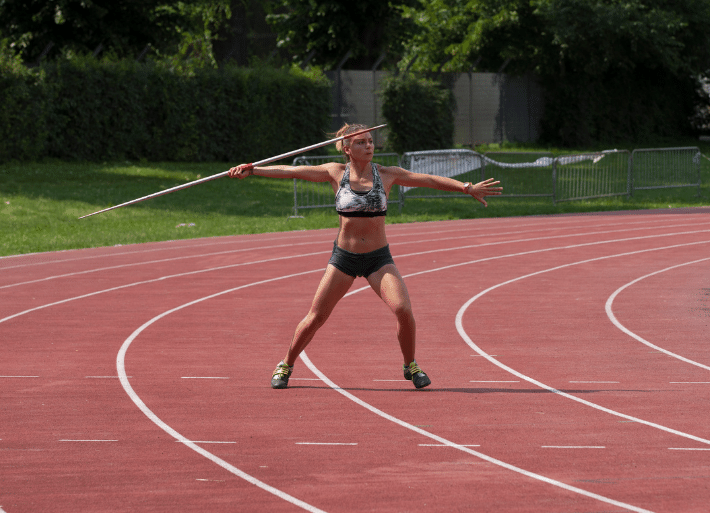This is a realistic, horizontally oriented photograph of a young white woman athlete on a standard oval-shaped red track and field track, made up of typical track material and marked with white lines separating the lanes. She is dressed in a black training shorts and a black, white, and gray training bra, along with athletic shoes. Her blonde hair is tied in a ponytail, and she is wearing a large watch on her left arm, possibly a smartwatch. The athlete is holding a white or silver metallic javelin with a red tip and a red handle in her gloved right hand, and she is captured mid-motion, seemingly about to launch it. The background features a green grassy field, taller shrubs, and a mix of green trees, as well as a chain-link fence and a metal barricade used for crowd control. There is no audience visible, focusing the attention solely on the determined athlete in action.